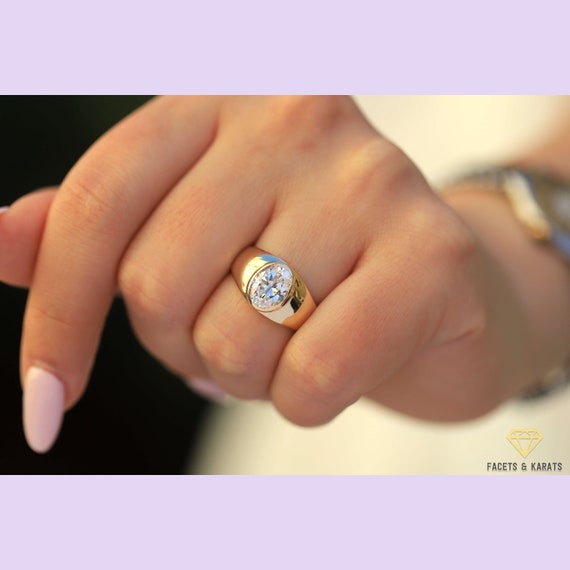The image features a highly detailed, close-up photograph of a woman's left hand, showcasing her wedding ring. The photograph is framed by thick borders in a delicate light purple or lavender hue at the top and bottom. In the center, the photograph captures the woman's clenched fist, with her forefinger extended, revealing long nails painted in a pretty pink polish. The focus is on her ring finger, which is adorned with a thick gold band set with a prominent oval-shaped diamond. To the right side of the image, her wrist and arm extend out of focus, and a blurred silver and gold watch can be seen. The background to the left of the hand is solid black, while the middle and right side feature an ivory backdrop, possibly indicating the woman's dress. In the bottom right corner, there is a yellow-outlined gem with the words "FACETS" and "CARATS" written beneath it in small, all-caps, black text.